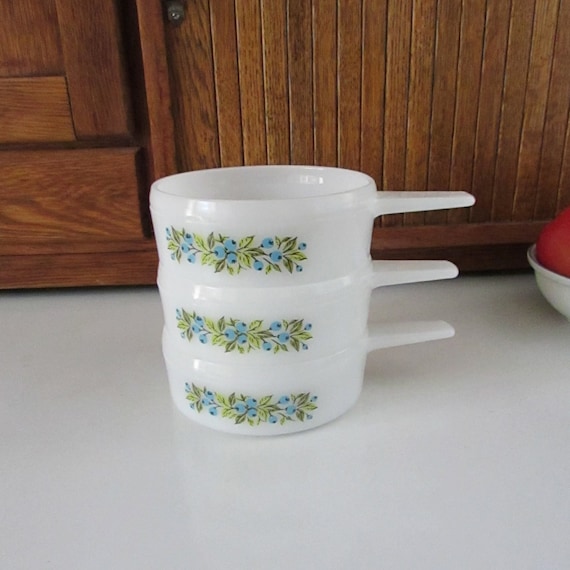The photograph, captured in an indoor setting, showcases three white ceramic measurement cups stacked on top of one another on a plain white countertop, likely made of formica. Each cup features a flat handle extending from its right side and is adorned with a decorative pattern of green leaves interspersed with clusters of light blue blueberries, each dotted in dark blue, spanning horizontally across the cups. The countertop is part of a room characterized by brown wooden cabinetry in the background. Additionally, to the right side of the frame, partially visible, is a white oval-shaped bowl with a red lid. The overall scene is set against the backdrop of the sleek, minimalist kitchen decor.